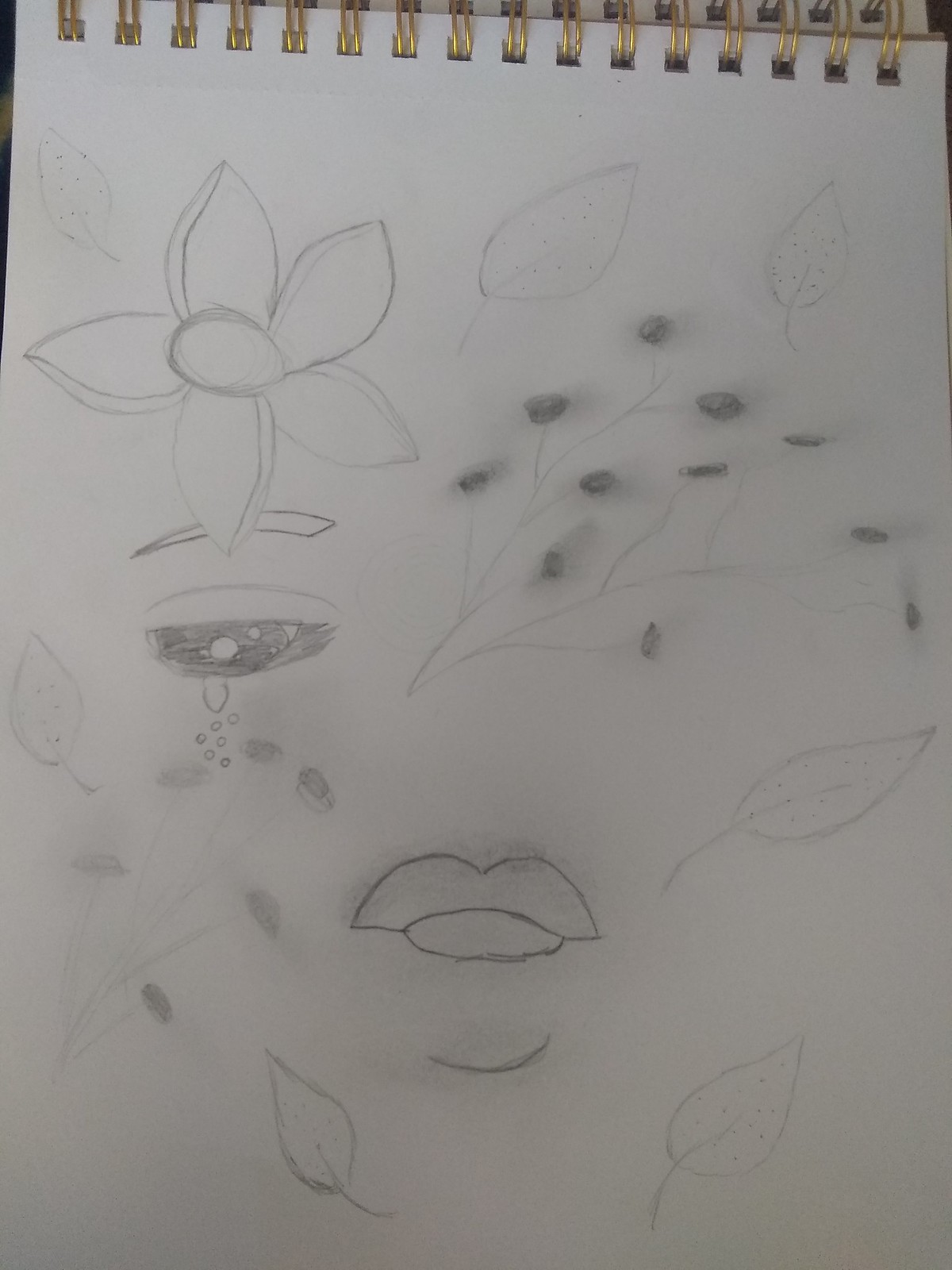A detailed pencil sketch occupies a page in a spiral-bound, gold-spiraled sketchbook. At the center of the composition is a single, expressive eye shedding a tear. Above the eye, a finely detailed eyebrow arcs gracefully, while a delicate flower blooms above it, surrounded by intricately drawn leaves. Various additional leaves and what appear to be clusters of berries are scattered around the scene. Below the eye, a slightly open mouth is depicted, revealing a hint of emotion. A fragment of a chin peeks out from beneath the mouth, contributing to the impression of a partial face enveloped in an organic arrangement of leaves and a single blossom. The monochromatic pencil drawing captures a blend of human and natural elements in a hauntingly beautiful manner.